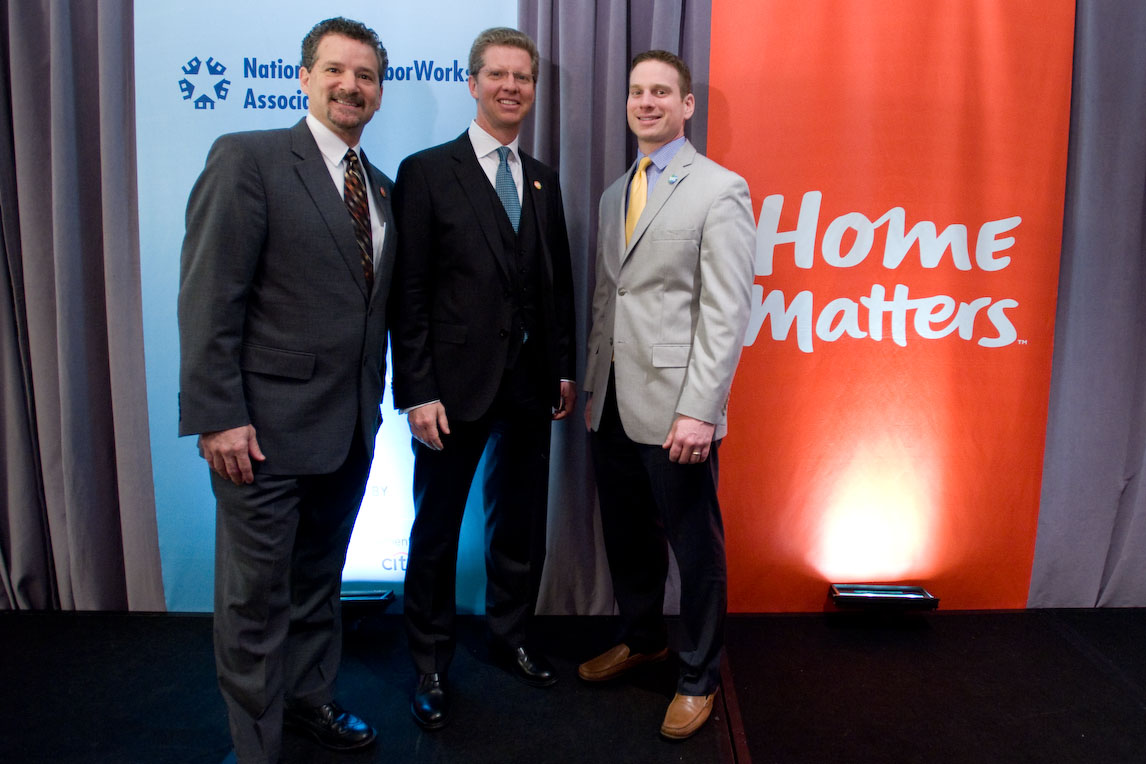This business photograph captures three middle-aged men standing in front of two prominent background banners at what appears to be a professional convention, likely for a work magazine or news article. All three men are dressed in formal attire, wearing dress pants, dress shoes, button-down shirts, ties, and suit jackets, and they are all smiling warmly at the camera. The man in the center is distinguished by his black suit, white shirt, blue tie, and a small gold pin on his lapel. To his right, another gentleman is in black pants, brown shoes, a light tan dress jacket, a blue button-up shirt, and a yellow tie. On the left, the third man sports gray dress pants, black shoes, a gray jacket, a white button-up shirt, and a black multi-colored tie. One of the men also has a mustache, adding a distinctive touch to his appearance.

They are positioned in front of two clear banners and a gray curtain backdrop, which is subtly illuminated, enhancing visibility. The orange banner with white text reads "Home Matters," while the other, light blue with blue writing, partially legible, likely states "National Labor Works Association." The black floor beneath them adds contrast to the image, and their hands rest casually at their sides as they confidently present themselves, adding to the formal yet welcoming atmosphere of the photo.